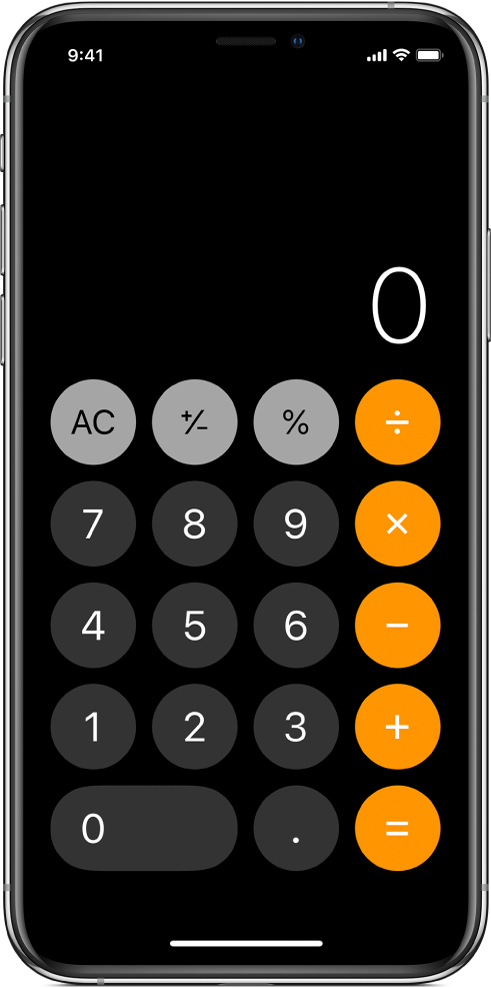The image features the interface of a tablet or smartphone, with the top left corner displaying the time "9:41." On the top right, there are two small blue circles, four signal bars, a Wi-Fi icon, and a full battery indicator. The background beneath this status bar is black.

Toward the middle right of the screen, there is a prominent white "0." Below this, to the left, is a gray oval labeled "AC." To its right, there's another gray oval with a plus sign, a slash, and a minus sign. Further to the right, another gray oval displays a percent sign. Adjacent to it on the right is an orange oval with a division icon.

In the following row, there are gray ovals with the numbers "7," "8," and "9" sequentially. To their right, there's an orange oval featuring an "X" symbol.

The subsequent row contains more gray ovals with the numbers "4," "5," and "6." The oval on the far right is orange and bears a minus sign.